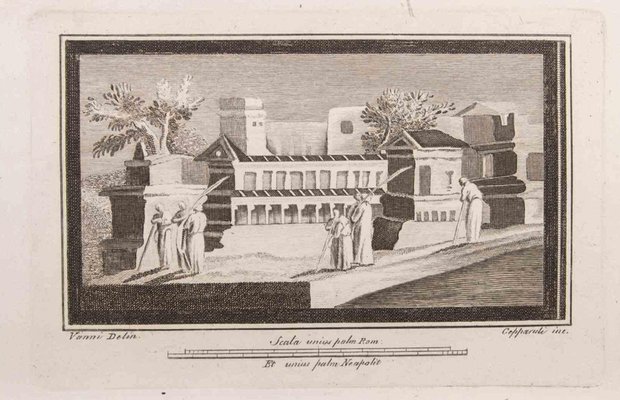This detailed black and white lithograph depicts an ancient or Romanesque scene, framed by an aged, cream-colored parchment bordered by two dark lines. The central image showcases a group of people engaged in agricultural work, likely tilling or planting a garden. In the foreground, three individuals wield gardening tools, while three more are positioned slightly to the right, and another person tends to the ground in the background.

The figures are clad in robes resembling cloaks and are holding elongated implements, which could be shovels, brooms, or large feathers. The backdrop features a series of old buildings: a prominent white house with numerous small windows, a distinctive watchtower-like structure, and a sectioned dark roof accentuated by white lines. Additionally, there are indications of irrigation with streams of water flowing from small structures flanking the garden, suggesting advanced agricultural techniques of the time.

Tiny, highly stylized cursive writing adorns the bottom of the page, though it remains illegible. The scene is complemented by trees scattered throughout, including one oddly positioned atop a high roof, adding a touch of surrealism to the otherwise historical setting. To the far right, there is a body of water, likely a lake, pond, or seashore, adding a serene element to the industrious scene.